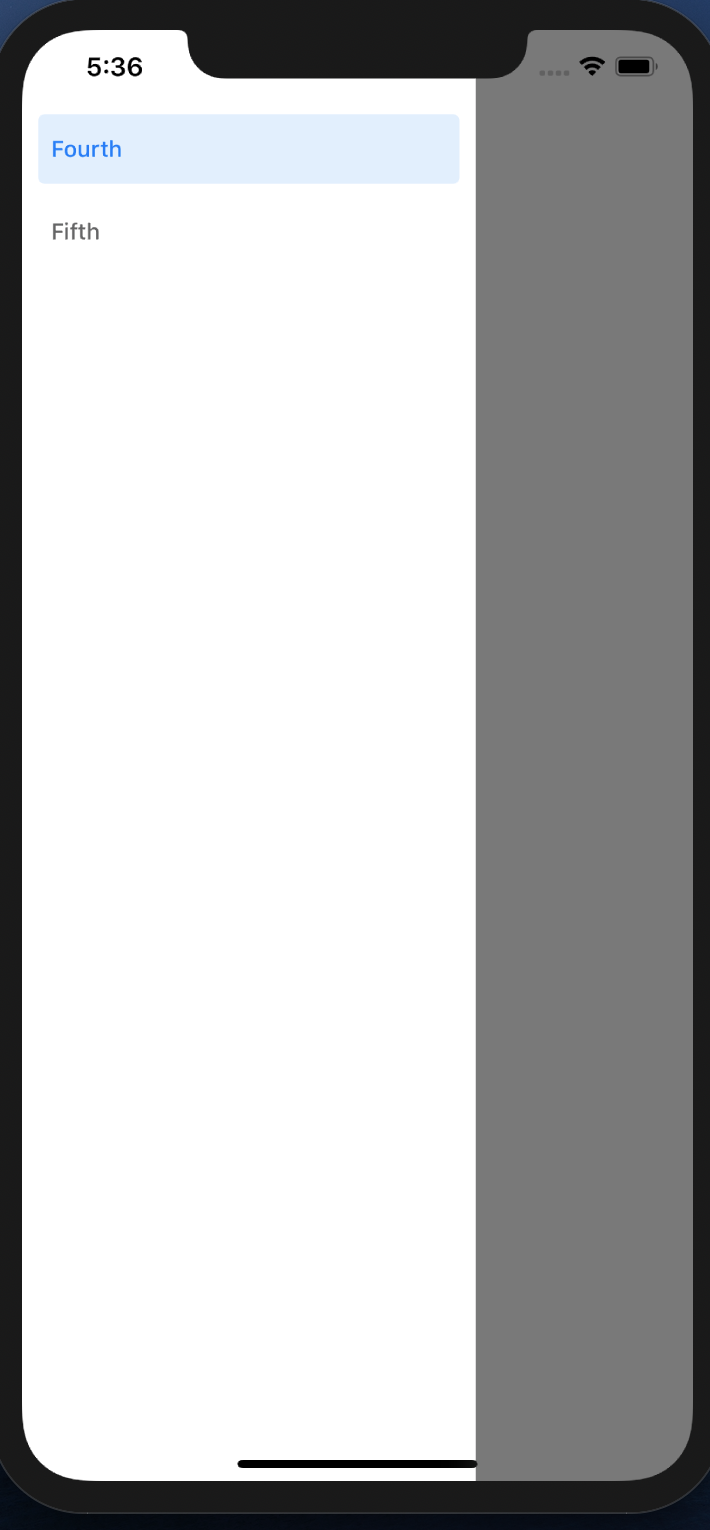The image displays a minimalistic app interface, likely on an Apple device due to its design elements distinct from Android. The screen is divided into two unequal sections; the left two-thirds is bright while the right one-third is slightly darker, indicating an option has been selected or tested. The interface prominently features two date options, "4th" and "5th," with "4th" highlighted in blue. In the upper left corner, the time is displayed as 5:36, although it is unclear if this represents AM or PM. A thin line spans a third of the screen towards the middle, further suggesting this could be a prototype for an app or a feature in development. The overall color scheme is black and white, emphasizing the minimalist design aesthetic.